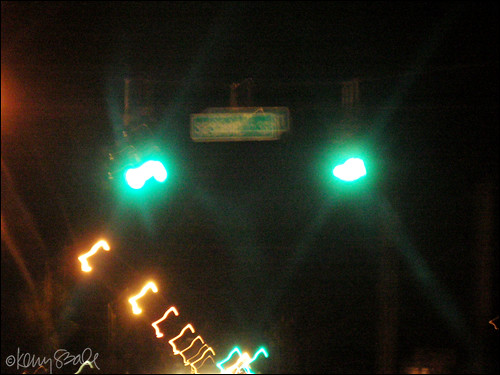This nighttime photograph captures a blurred and distorted scene. Central to the image are two green lights, likely traffic lights or stage lights, positioned symmetrically with one to the left and the other to the right of center at the same height. Suspended between these lights is an unreadable, blurry white sign. Additionally, the bottom left corner features a diagonal, L-shaped light trail, suggesting a time-lapse effect, descending from the center of the bottom-left quadrant to the bottom-middle of the frame. Also in the bottom left corner, there's a cursive watermark, presumably the artist or photographer's signature, which is difficult to read due to its scribbled nature.